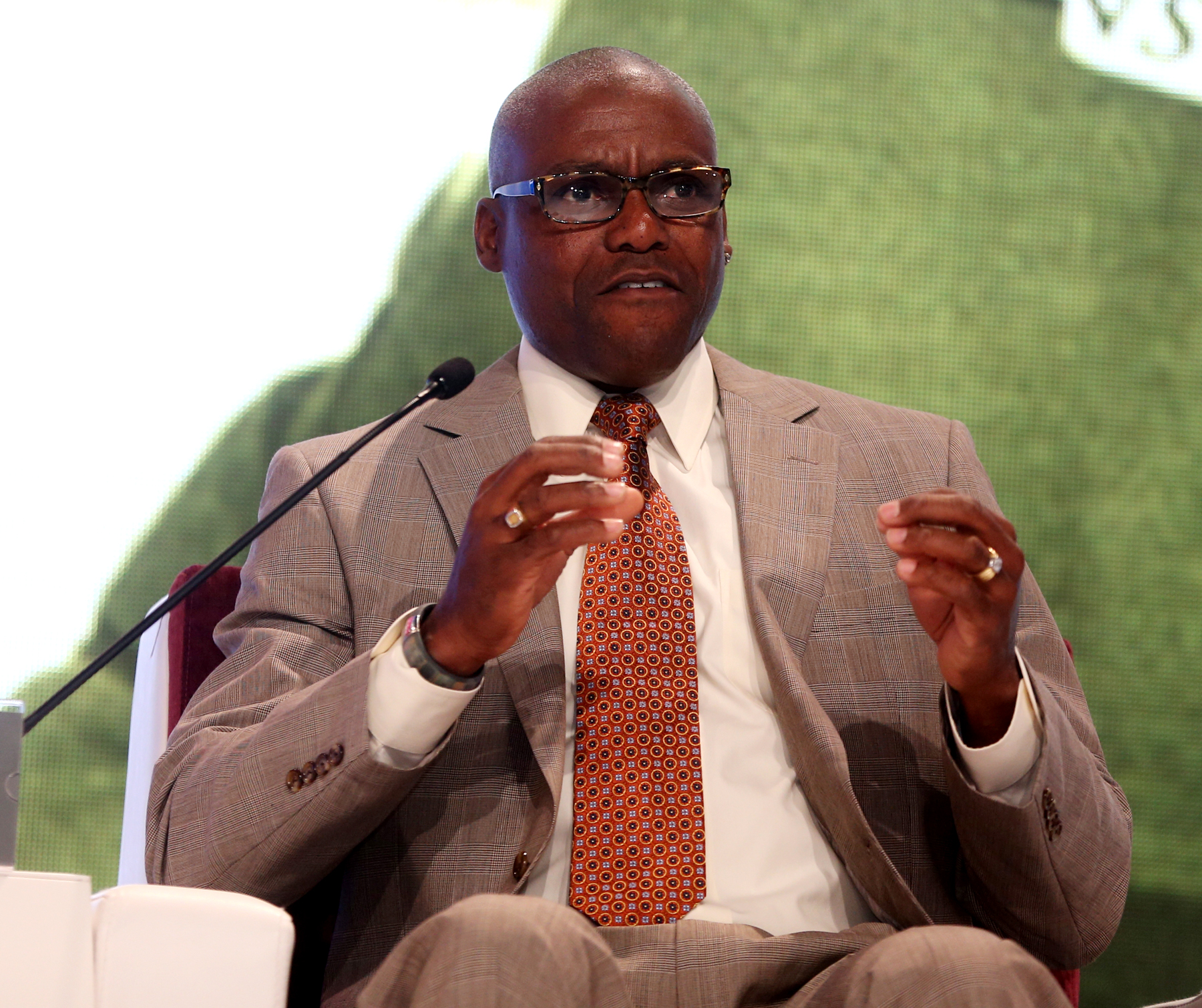A black, middle-aged, bald man is seated on a white leather upholstered chair with a red plush cushion on the backrest, positioned on a stage. He is dressed in tan-colored dress pants and a gray, striped business coat with four buttons on each sleeve. Underneath, he wears a button-up white dress shirt paired with a red tie adorned with multiple orange and black circles. The man, who also sports brown-framed glasses and a studded earring in his left ear, appears to be addressing an audience, with his upper teeth visible and a thin black stand microphone angled towards his face from the left side. He is wearing rings on both his ring fingers and a wristwatch on his right wrist. The background comprises an LED screen radiating a design that prominently features a large green shape.